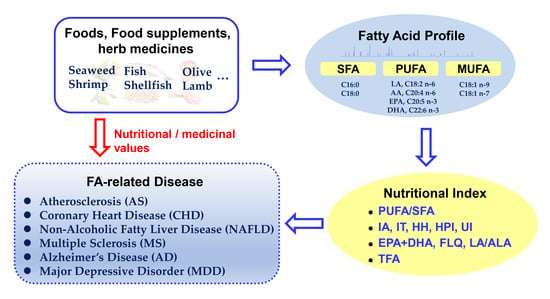The image depicts a detailed diagram outlining the relationship between various food items and their nutritional and medicinal implications. The diagram is divided into four interconnected sections. 

In the top left, a white rectangle with a blue border is labeled "Food, Food Supplements, Herb Medicines," listing items such as seaweed, shrimp, fish, shellfish, olive, and lamb. An arrow from this section points to the upper right, connecting to a light blue circle labeled "Fatty Acid Profile," detailing SFA (Saturated Fatty Acids), PUFA (Polyunsaturated Fatty Acids), and MUFA (Monounsaturated Fatty Acids). 

From the blue circle, a blue arrow points downward to a yellow oval titled "Nutritional Index," which includes numerous acronyms such as PUFA/SFA, IA, IT, HH, HPI, UI, EPA + DHA, FLQ, LA/ALA, and TFA, indicating various nutritional metrics.

Both the "Food, Food Supplements, Herb Medicines" rectangle and the "Nutritional Index" oval direct to the final section, a blue rectangle labeled "FA-Related Disease," listing diseases like atherosclerosis, coronary heart disease, non-alcoholic fatty liver disease, multiple sclerosis, Alzheimer's disease, and major depressive disorders. Additionally, this blue rectangle has a red arrow pointing to it labeled "Nutritional/Medicinal Values," summarizing the overall focus of the diagram.